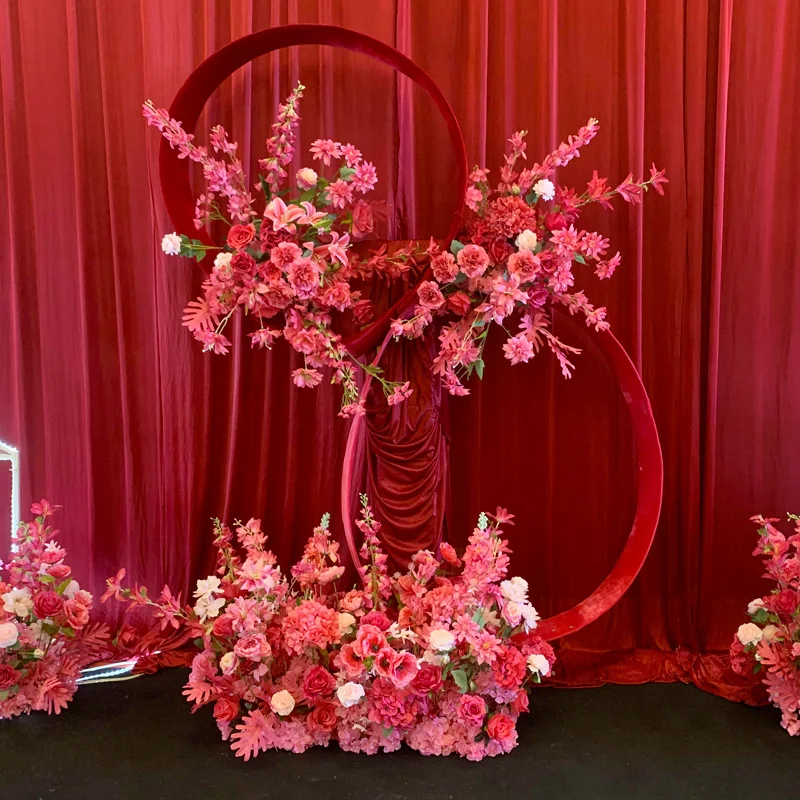The photograph features an intricate floral arrangement on a black floor, set against a backdrop dominated by a rich red curtain. Central to the arrangement is a vase housing primarily pink and red roses, supplemented by a scattering of white flowers. A red fabric-wrapped column runs up the middle, flanked by two substantial floral structures with corresponding large, circular loops—one around the left structure and a larger, partial loop around the right.

Towards the bottom of the image, three main clusters of flowers are arranged, with additional bunches on either side peeking into the composition. The leftmost and rightmost thirds of the image display additional red flowers, adding to the overall complexity. Overall, this setup has a grand, almost sculpture-like feel, with the flowers intricately layered and meticulously placed, creating a vivid and dynamic floral design.